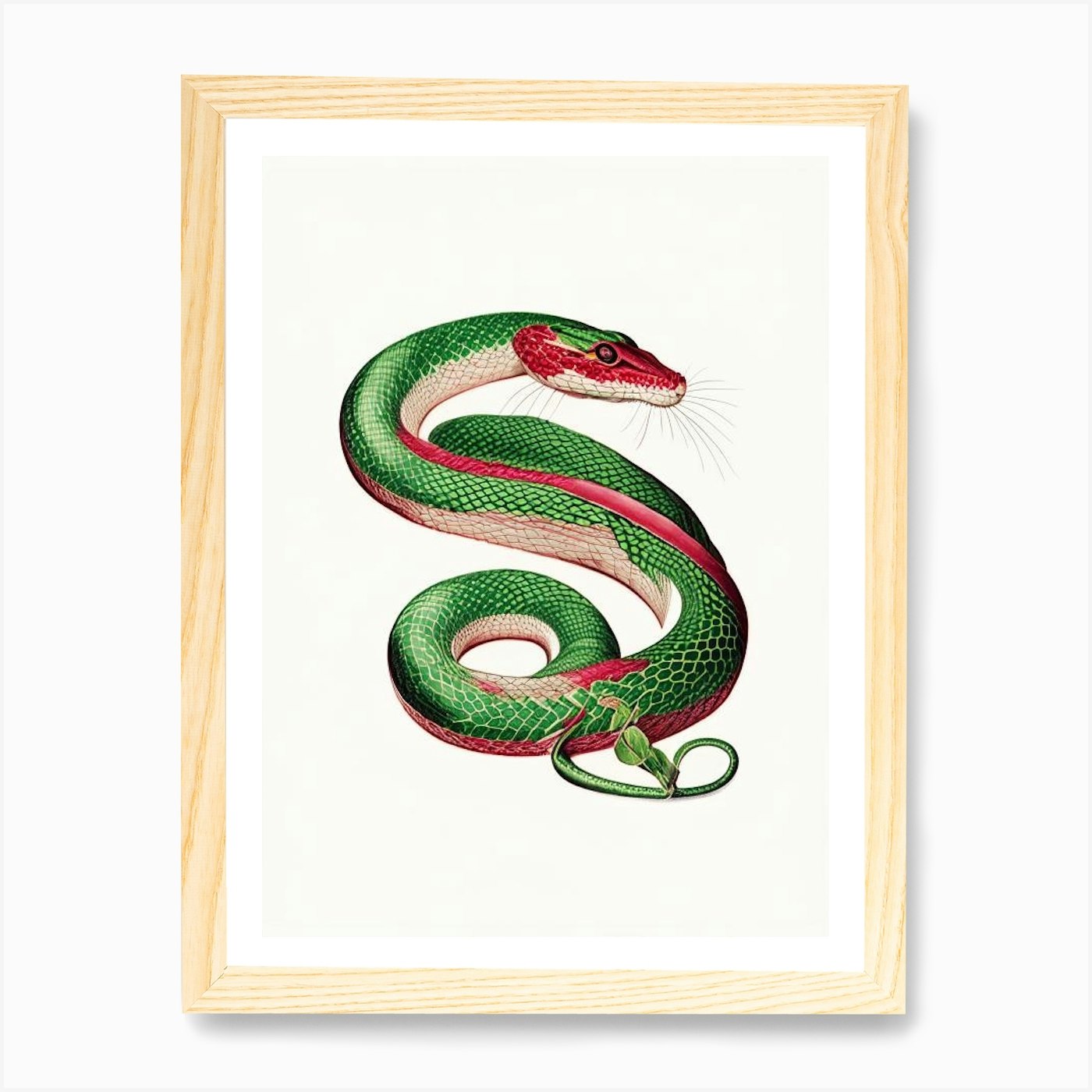The image depicts a framed artwork centered on a white background devoid of other elements. The piece is enclosed in a light brown, thin wooden frame showcasing natural patterns, casting a light drop shadow down to the right. Within this frame, a white mat border surrounds the artwork, which is set against a beige paper background. The subject of the artwork is a realistically rendered yet colorfully stylized snake. The snake, oriented with its head facing right, adopts an S-curve positioning. The upper part of its head is vivid red, transitioning to white below the face, adorned with several whiskers. Behind its eyes, the green hue continues down the top of the body, consisting of alternating dark and light green scales. The bottom half of the snake's body is white, interspersed with red highlights, giving it a watermelon-like appearance. Subtly detailed, the tail resembles a vine, adding to the artwork’s intricate nature.